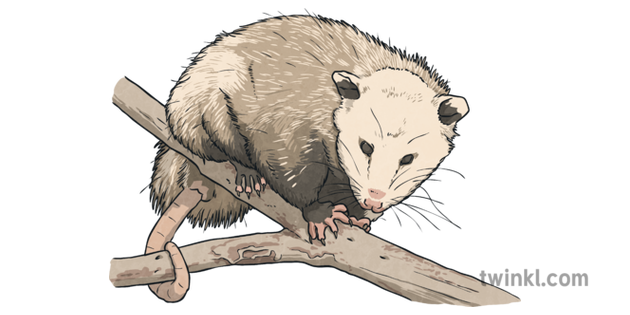The image is a detailed digital drawing of a possum perched on a light brown, textured branch that splits into a Y-shape near the center of the scene. The possum, with its white face, dark brown-black eyes, and ears, has a mix of white, light tan, and gray fur covering its body. It has a distinctive pink snout and mouth adorned with numerous black whiskers. The possum's positioning shows its back end to the left and its head to the right, seemingly facing the viewer. It uses its claws to grip the branch where it forks, with its right foot on the upper-left segment and its tail wrapped around the lower-left segment. The background is completely black, emphasizing the possum and the branch. In the bottom right corner, the watermark "twinkl.com" is displayed in gray letters, validating the source of the image.